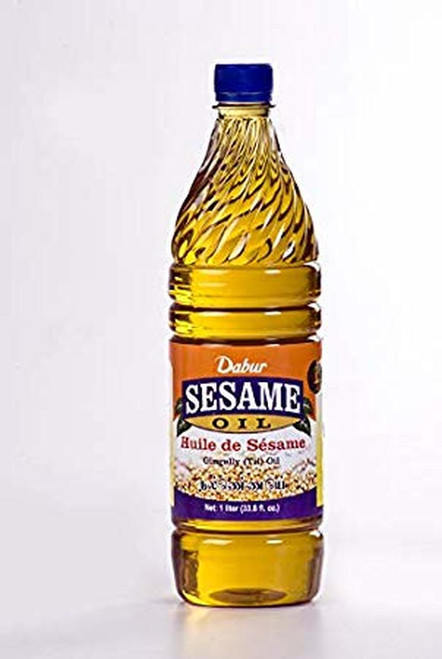The photograph showcases a clear bottle filled with light yellow sesame oil, set against a gradient background that transitions from a whitening gray on the right to a darker gray on the left. The bottle, standing on a flat gray surface, casts a visible shadow around its base. It features a blue cap and is similar in shape to a water bottle. The label, occupying the bottom half of the bottle, is multicolored with an orange upper segment. In the orange section, white text reads "Dabur". Below that, there is a white oval containing an image of a plant, and a blue banner with the white text "Sesame". Additional red text, reading "Huel de sesame," appears beneath it. The label informs viewers that this is a bottle of sesame oil, providing details about the product's name and fluid contents. The promotional image highlights the bottle's clear design, allowing the reflective, yellowish liquid within to be seen distinctly.